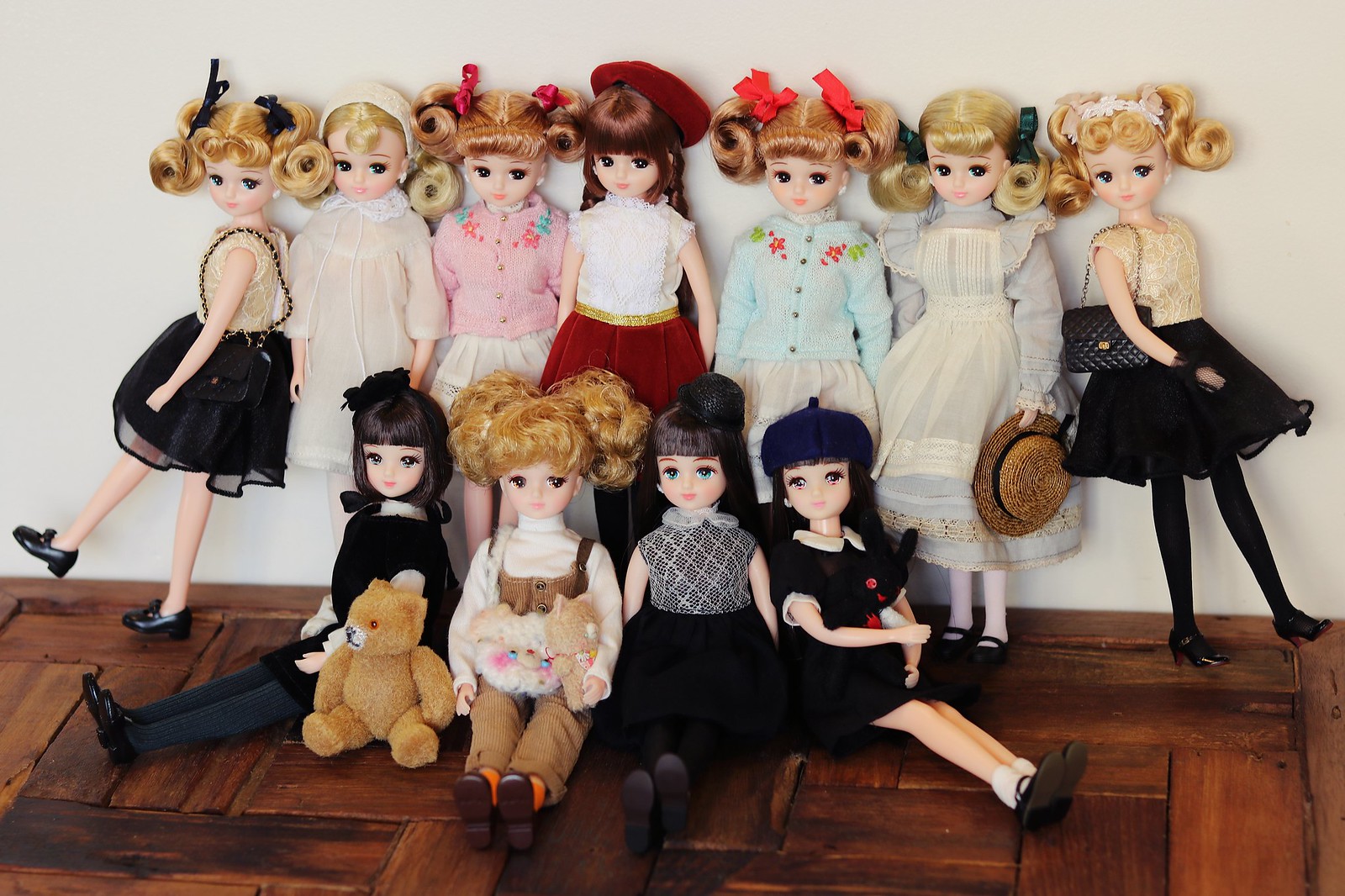This is a detailed photo featuring eleven vintage baby dolls, possibly from the 1930s, 40s, or 50s. The dolls are arranged on a dark brown, mahogany-colored wooden floor against a solid black wall. In the back row, seven dolls are either standing or propped up against the wall. Most of these standing dolls have blonde hair, with one exception featuring long brownish-red hair. Notably, the sixth doll in this row is holding a fashionable hat. In front of these standing dolls, four dolls are seated. Of these seated dolls, three have dark hair, while one has blonde hair. Each doll is dressed in a charming outfit consisting of a dress or a skirt paired with a colorful top. Their hairstyles vary, often featuring beautifully curled ends and bangs, accented with bows and ribbons. Adding to the scene, one of the seated dolls on the far left is holding a small teddy bear.